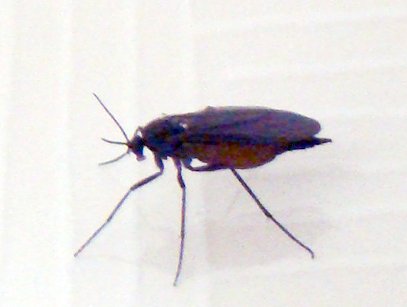The image shows a close-up of a small beetle-like bug, likely less than an inch long, standing on a white background that has faint lines resembling paper or a curtain. The beetle has a distinctive appearance with an oval-shaped, flat top that appears black or purplish depending on the lighting. Viewed from the side, its stomach area is visible and shows an orange to reddish hue. The bug has a tiny head with three slender antennae and a small, downward-facing posture. It has three stick-like legs that are brown to black in color and seem firmly planted on the ground. Additionally, it features a small tail-like structure at its rear. The beetle is oriented facing to the left in the image.